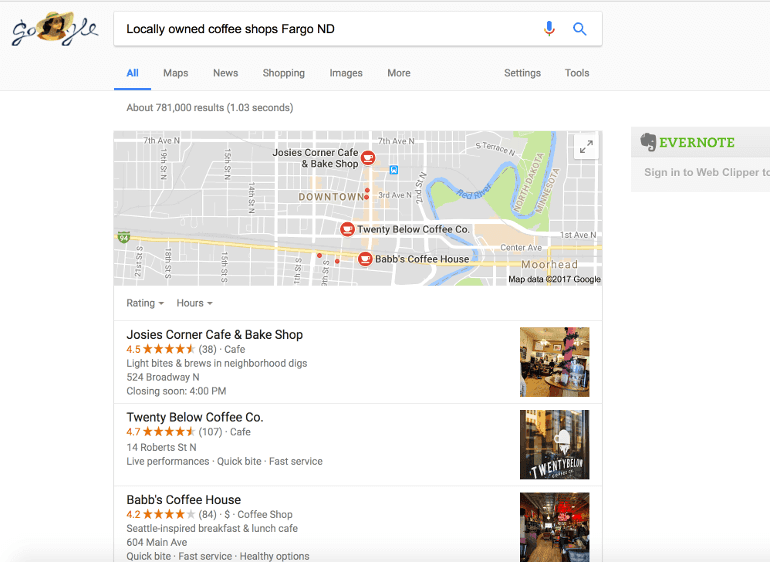Screenshot Description:
The image is a screenshot of a Google search results page. At the top, there is a light gray rectangle extending horizontally. In the upper left-hand corner of this rectangle, "G-O" is written in gray cursive letters. Adjacent to this, there is a small image of a woman with dark hair wearing a sun hat. Following the image, the letters "G-L-E" appear in the same gray cursive font, completing the word "Google." 

To the right of the Google logo, there is a white rectangular search bar. Inside the search bar, bolded in black text, is the query: "locally owned coffee shops, Fargo, ND." On the far right of the search bar, there are icons of a blue and red microphone and a blue magnifying glass.

Below the search bar, there is a menu bar with various options. From left to right, the options are: "All" (which is blue and underlined to indicate it is the selected filter), followed by "Maps," "News," "Shopping," "Images," and "More." On the extreme right of the menu bar are "Settings" and "Tools," written in gray.

Underneath the menu bar, there is a section that appears to be Google Maps integrated within the search results. This section lists three local coffee shops, each in its own separate rectangle. The listed establishments are:

1. **Josie's Corner Cafe and Bakeshop**
2. **20 Below Coffee Co.**
3. **Babs Coffeehouse**

Each coffee shop's name is bolded in black. To the right of each name, there is a square picture depicting the interior of the respective establishment. Below the name and image, each listing includes:
- A star rating
- A brief description
- The address
- The hours of operation